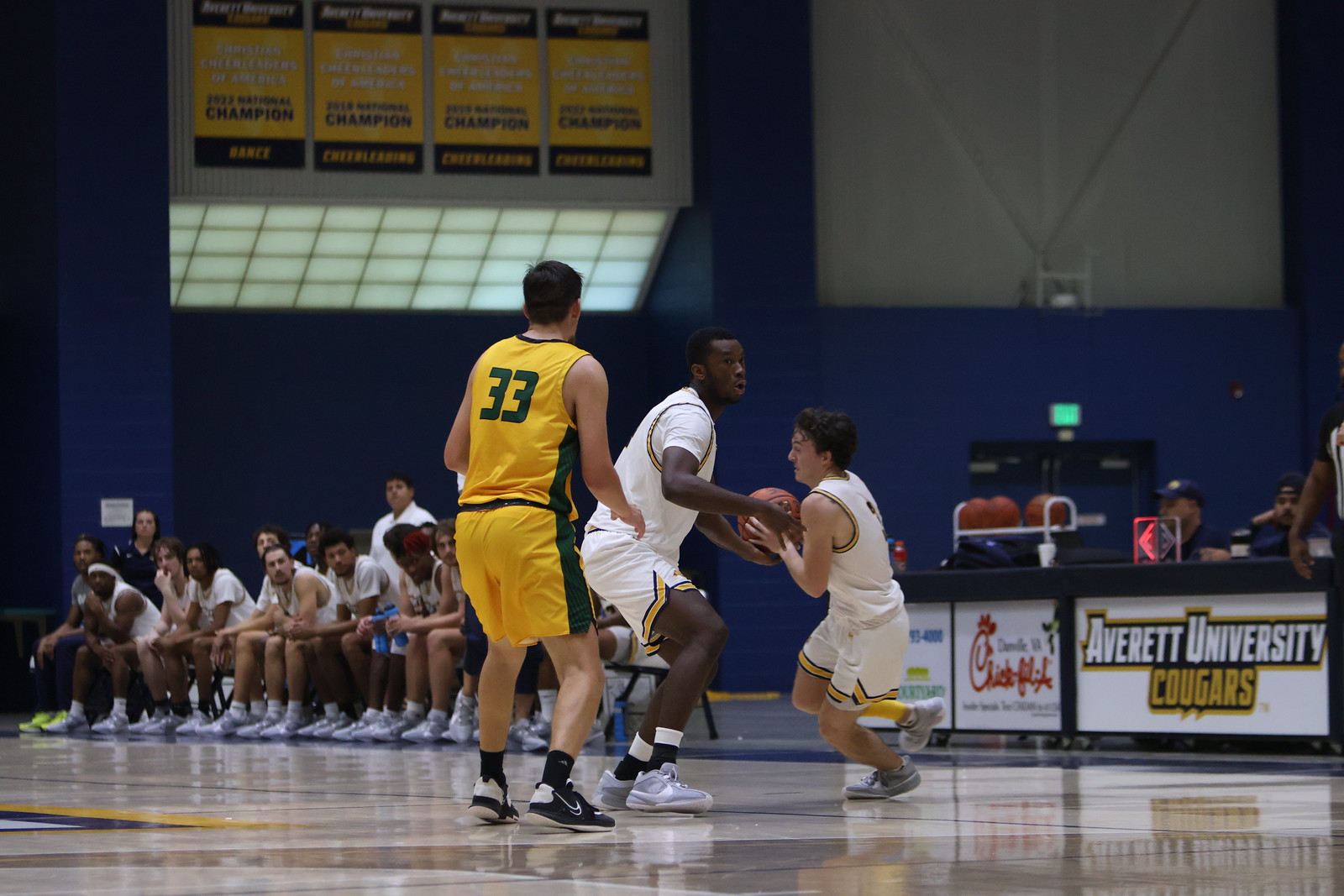In this detailed image of a live basketball game, two players are prominently attempting a ball handoff on the court. The first player is a taller black athlete in a white uniform with a white T-shirt underneath, gray sneakers, black and white socks, and looking off to his right. He appears to be passing the ball to a much shorter white player, also in a white uniform, who has his hands firmly on the ball. This shorter player is distinguished by gray sneakers and a yellow brace on his right leg. 

Standing with his back to the camera is an opposing player in a yellow uniform with green numbers and trim. His jersey number is 33, and he is wearing black socks and black sneakers. This player is white and appears to be preparing to intervene in the ball handoff.

In the background, the bench lined with about a dozen players from the white team is clearly visible, with a couple of individuals standing behind it, engrossed in the game. To the right of the bench is the scorer's table displaying a sign that reads “Averitt University Cougars” in white and gold lettering. The possession arrow illuminated on the table is pointing to the left, and three basketballs rest in a rack nearby.

The indoor gym features blue walls, a green exit sign above a door, high frosted windows, and several banners hanging high up, commemorating past championships. Additional details include a large white panel on the right side of the gym wall.